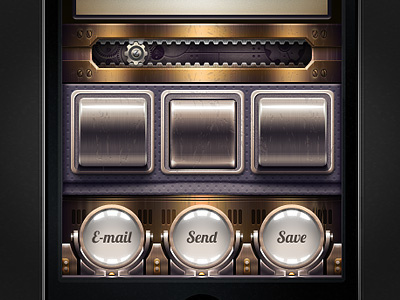The image is designed in a landscape orientation, resembling a steampunk-themed slot machine. Both the left and right edges feature a gray line that transitions into a silver strip, followed by a dark black strip. The central section has a faint off-white or light gray line with a silver line beneath it. Below this, there's a visible gear mechanism with silver teeth set against a gray background, encased in a gold frame with matching gold screws.

At the bottom of the image are three circular, glass-like buttons framed in silver. The left button says "E-Mail" in black cursive text, the center one says "Send" in black, and the right button says "Save" in black. These buttons are set against a dark background.

Above these buttons are three square sections that appear like the rollers of a slot machine, silver in color with varying shades of gray behind them. Higher up, there's an open slot area featuring a horizontal-moving gear, also silver, surrounded by a metallic bronze or gold color. The overall design combines both visual elements of a slot machine and intricate, mechanical details, contributing to a steampunk aesthetic.